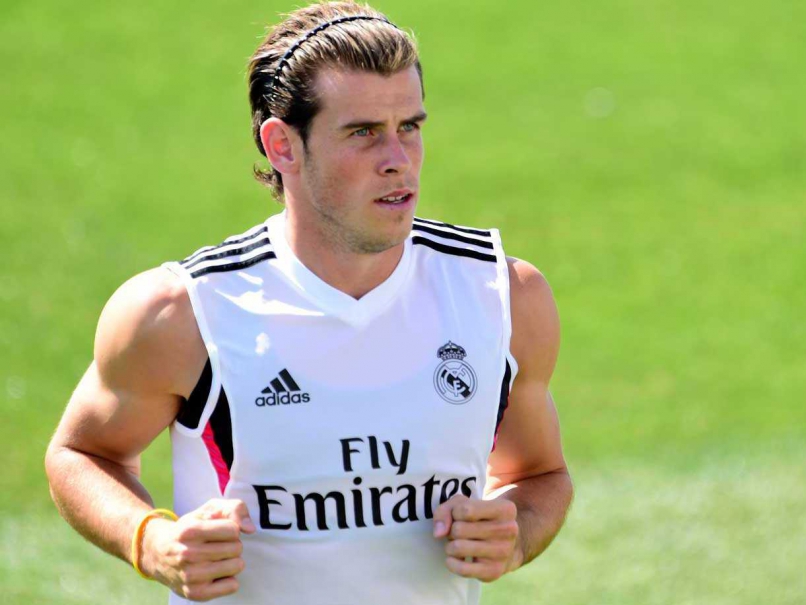The photograph captures a male athlete jogging on a grassy field. The athlete, visible from the chest up, has medium-length hair pulled back with a black headband. He is dressed in a white jersey adorned with dark stripes on the shoulders and dark accents. Prominently displayed on the front of the jersey is the text "Fly Emirates" in black, with an Adidas logo located above it. A second, partially visible logo appears to be a circular emblem featuring a crown and possibly the letters F, C, and M, hinting at a football club affiliation. The athlete has both fists clenched and is wearing a yellow wristband on his right arm. His muscles are visibly tensed, and his arms are raised to the level of his ribs. The background is blurred, highlighting the green grassy field he is on.